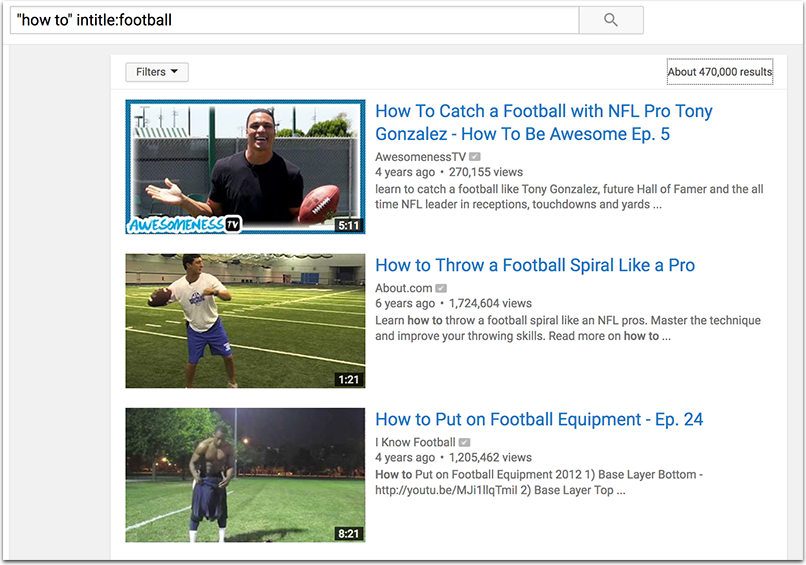The image portrays a search results page with the following details:

- At the top left of the image, there is a search bar displaying the query "how to" in quotation marks, followed by the word "entitled: football." To the right of the search bar, a gray button with a magnifying glass icon is present, indicating the search function.
- The background beneath the search bar is primarily gray. It features a narrow gray area at the top and on the right side, while the left side has a wider gray section.
- Below this gray section, there is a white box comprising several components:
  - A drop-down menu labeled "Filters" located at the top left.
  - An indicator on the top right showing "About 470,000 results."
- The content below this area includes several search results which feature thumbnails and descriptions:
  - The first result is a thumbnail of a man holding a football and smiling at the camera. The video duration is noted as 5 minutes and 11 seconds. The title reads, "How to Catch a Football - NFL Pro Tony Gonzalez, How to Be Awesome Episode 5."
  - The next result to the left features a thumbnail of a man throwing a football. The video duration is 1 minute and 21 seconds. The title is "How to Throw a Football Spiral Like a Pro."
  - Under these results, another video is shown with a thumbnail of a man on a football field. This video is titled "How to Put on Equipment - Episode 24, Football Four Years Ago."

This detailed description encapsulates the visual and textual elements observed in the search results page.